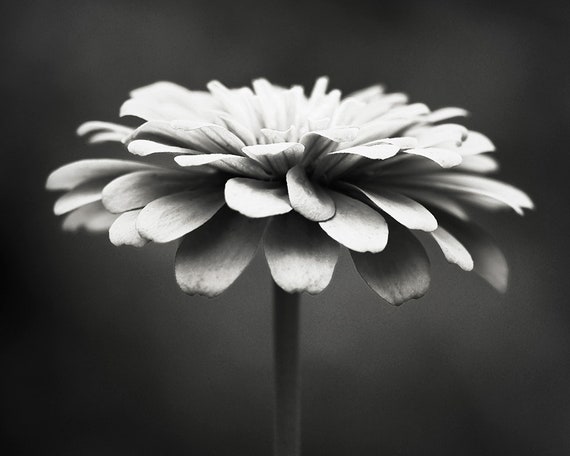The black-and-white photograph showcases a solitary flower with a single stem, surrounded by a hazy, indistinct background created by a bokeh effect, giving the impression that the flower exists in a vacuum. The composition centers around the flower, displaying a direct, straight-on view that is perfectly symmetrical, emphasizing its round shape reminiscent of a plate. The petals, small and closely arranged, flare out in tiers without pointed tips, appearing flat at their ends. The petals exhibit darker veining or shading, indicating texture and depth, hinting at their original, likely bright color. This artistic capture, possibly of a daisy or marigold, is defined by the striking light and dark contrasts, making the flower's delicate structure and inherent beauty the focal point of the image.